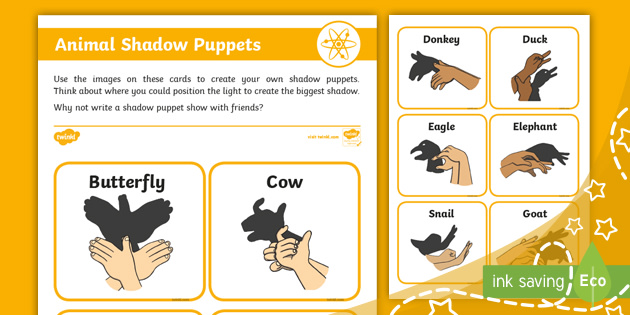The infographic, likely from a child's magazine or camp guide, prominently features the creative activity of making animal shadow puppets with hands. At the top, against an orange background, bold white text reads "Animal Shadow Puppets." Directly beneath, in black text on a white background, it instructs, "Use the images on these cards to create your own shadow puppets. Think about where you could position the light to create the biggest shadow. Why not write a shadow puppet show with friends?"

The infographic is divided into different sections, showcasing examples of shadow puppets. In the bottom left corner, there is an illustration of hands creating a butterfly shadow, labeled "Butterfly." Next to it, another set of hands forms a cow shadow, with the label "Cow" above. The right side of the infographic features more examples with labels for various animals like "Donkey," "Duck," "Eagle," "Elephant," and "Snail." Although the "Goat" example is partially obscured by an overlay, its label is still visible. These examples are drawn or digitally illustrated to demonstrate the hand positions and the corresponding shadows.

In the bottom right corner, a green section stands out with white text that reads "Ink Saving Eco," highlighting an eco-friendly aspect of the infographic. The word "Eco" is prominently written in a teardrop shape. Overall, the infographic combines vibrant visuals and detailed instructions to engage children in the fun and imaginative activity of creating animal shadow puppets.